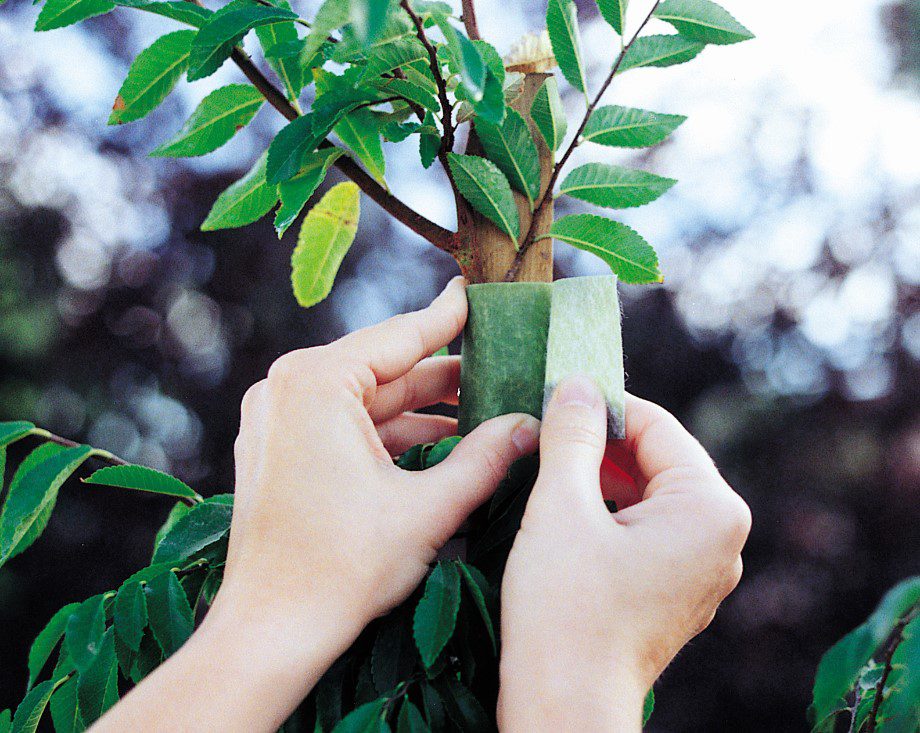This image captures an intricate scene of hands carefully tending to a young tree. The tree is slender, with a trunk approximately one to two inches in diameter and several small green leaves adorning its branches. A pair of delicate, likely Caucasian, and possibly feminine hands are seen wrapping a green, fibrous, possibly biodegradable tape around the tree. This tape, which resembles a textured fabric, appears to be providing support or perhaps mending damage to the tree. The tree is being tied to a wooden post, presumably to help it grow upright. The background of the image is artistically blurred, showcasing a bokeh effect with spots of bright white light filtering through, suggesting this scene is set outdoors, possibly in a garden or wooded area. The focus on the hands and the tree emphasizes the care and effort being put into nurturing the plant.